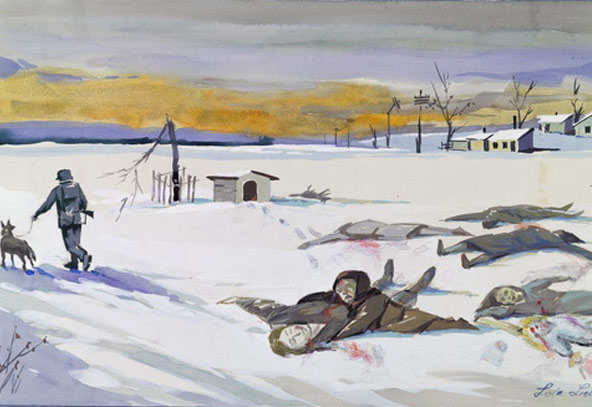This detailed and haunting illustration depicts a snowy, winter landscape under a somber sky tinged with green-gray, purples, and hints of yellow and orange. In the distance, bare trees and scattered houses break the horizon beneath a cloudy sky, while purple mountains loom in the background. The foreground is dominated by a heavy blanket of snow, marred by a gruesome scene of bloodied bodies with red holes in their chests or heads, suggesting a fresh massacre. Near the center-left, a doghouse with footprints leading away stands next to a broken tree enclosed in a small square fence. Nearby, a man dressed warmly in a winter coat, pants, and hat, carries a rifle and walks a German Shepherd on a leash. To the upper right, broken power lines add to the desolate atmosphere. This chilling image captures the aftermath of a violent event in a cold, eerily tranquil setting.